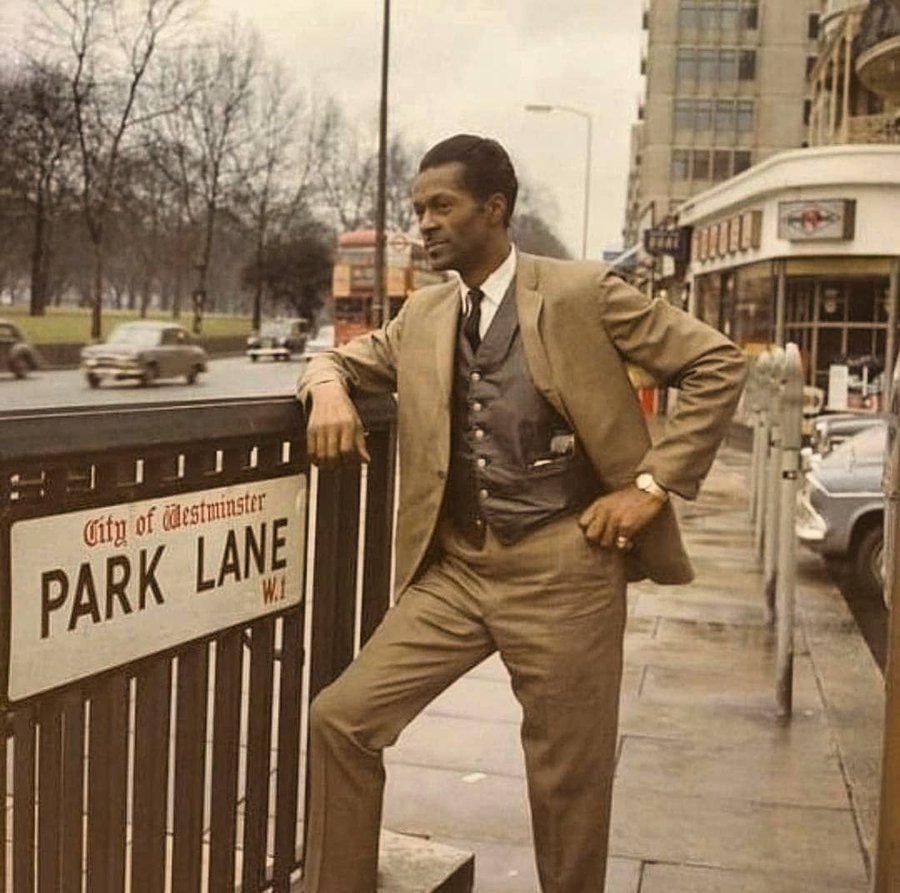In this meticulously detailed photograph, a sharply dressed Black gentleman stands on a sidewalk, evoking a sense of the 1950s or early 1960s. He's elegantly attired in a light brown suit jacket over a dark brown vest, paired with brown pants, a black tie, and a white collared shirt. His short, slightly combed-back hair complements his polished appearance, accentuated by a gold watch and a pinky ring on his left hand.

His right arm is poised on a waist-high fence—possibly wooden—adorned with a prominent sign that reads "City of Westminster" in red letters, with "Park Lane" in black, and the letters "W-I" in red beneath. The fence rests on a small, concrete step, adding a slight elevation to his stance.

The scene behind him is bustling with mid-century urban life. Over his right shoulder, a double-decker bus and a few European cars navigate the street, while to his left, more parked cars line the curb. A green park with trees stretches out across the road on his left, adding a touch of nature to the cityscape. On his right, the sidewalk extends past parking meters and leads towards a row of storefronts, with larger buildings rising further beyond. He stands with his left hand confidently on his hip, looking straight ahead with an expressionless demeanor, embodying the poised and timeless elegance of the era.